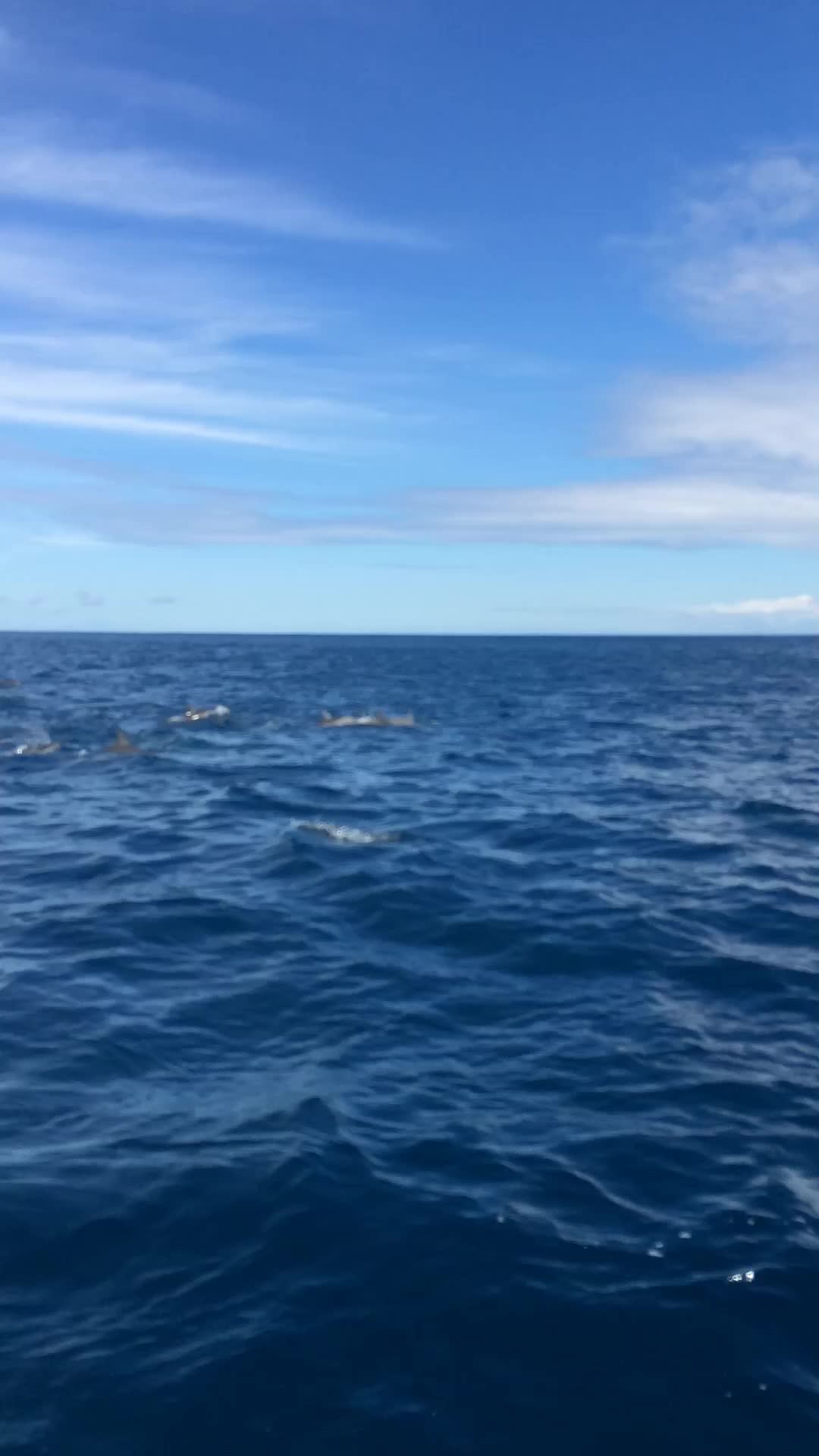This vertical, outdoor color photograph, taken in bright daylight, captures a vast expanse of the ocean and the sky. The lower half of the image showcases the ocean, characterized by its deep, dark blue water with a few white breaks, likely waves, breaking the surface. Near the middle and to the left, the water appears lighter blue and slightly blurred, indicating distant objects—possibly dolphins or porpoises—breaching the surface, though they are indistinct and out of focus. The horizon is flat and unbroken, devoid of any land features or text. The upper third of the photograph features a serene blue sky adorned with streaky white and gray clouds. The overall image is slightly blurry, giving it a sense of motion and immediacy, as if taken swiftly from a ship in an attempt to capture the elusive marine life below.